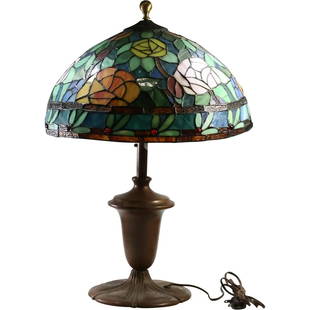The image showcases a single antique-looking table lamp positioned centrally against a white background. The lampshade, crafted from stained glass, features a green exterior adorned with ornate rose and flower patterns in multiple colors, giving it a vintage appeal. The dome-shaped lampshade is topped with a small circular piece. The lamp stands on a dark brown metal base, and a black cord emerges from the bottom right side of the lamp, running off the edge of the image. Overall, the lamp presents a classic, outdated aesthetic due to its stained glass design and antique characteristics.